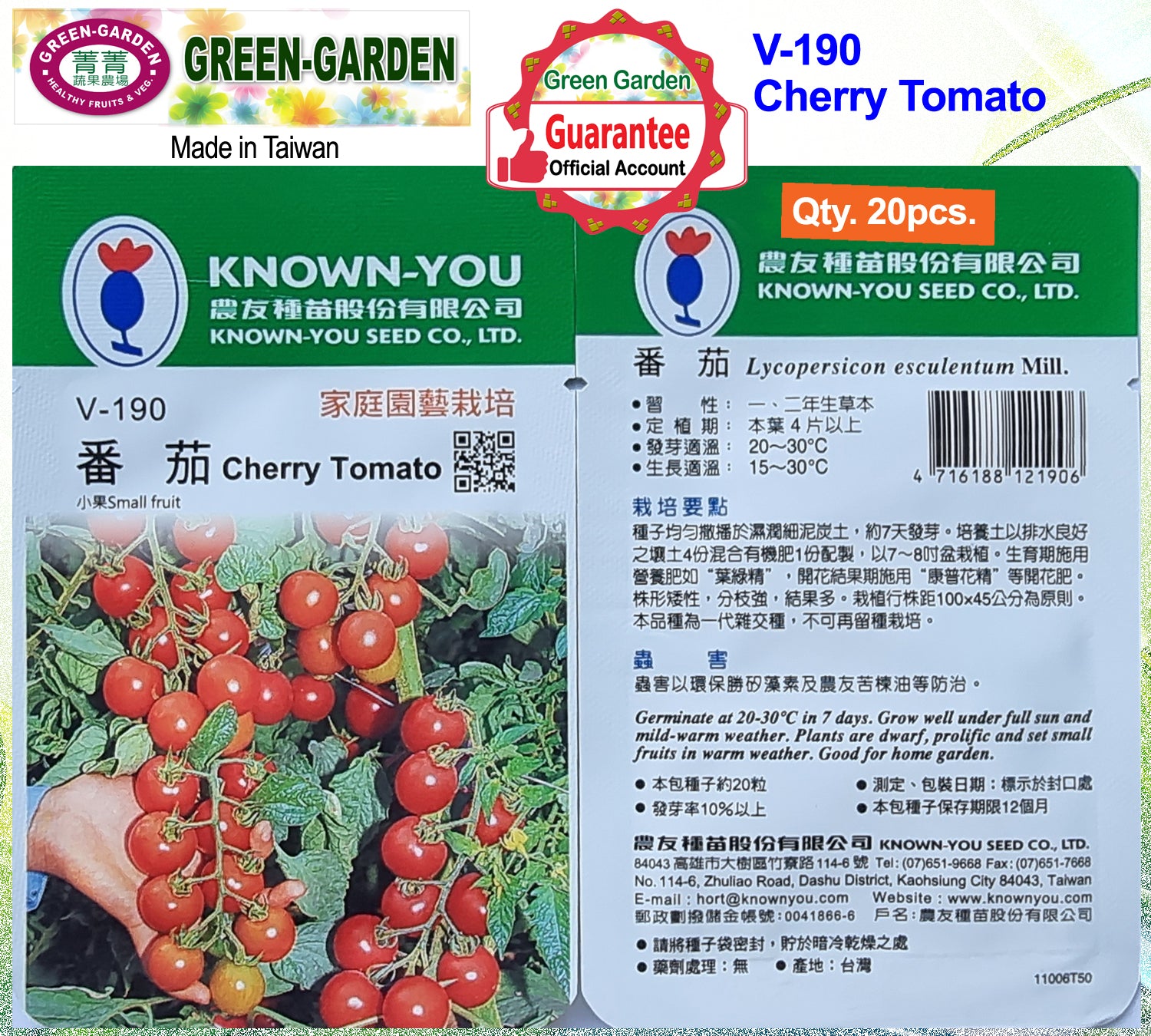The image depicts the front and back of a seed packet for V-190 Cherry Tomatoes from the Green Garden Company, made in Taiwan. The background of the packet is white, featuring a maroon oval at the top left that says "Green Garden" next to green capital letters also spelling "GREEN-GARDEN" against a backdrop of multicolored flowers. In the center at the top, there's a round red circle with a scalloped edge, indicating "Green Garden, Guarantee Official Account Inside." To the right, "V-190 Cherry Tomato" is written in blue. The top third of the seed packet is green and displays the company name, "No-Yu Seed Co., LTD," alongside Chinese text. A photograph of red, shiny cherry tomatoes on the vine appears at the bottom left, showing approximately 30 tomatoes. The right side of the packet is filled with extensive Chinese writing, but notable English details include growing instructions: the seeds germinate in 7 days at 20-30°C, thrive under full sun and mild warm conditions, and are suitable for home gardens due to their dwarf prolific nature. The packet specifies a quantity of 20 seeds and includes a barcode numbered 716188 121906. Additionally, the scientific name Lycopersicon esculentum Mill. is mentioned.